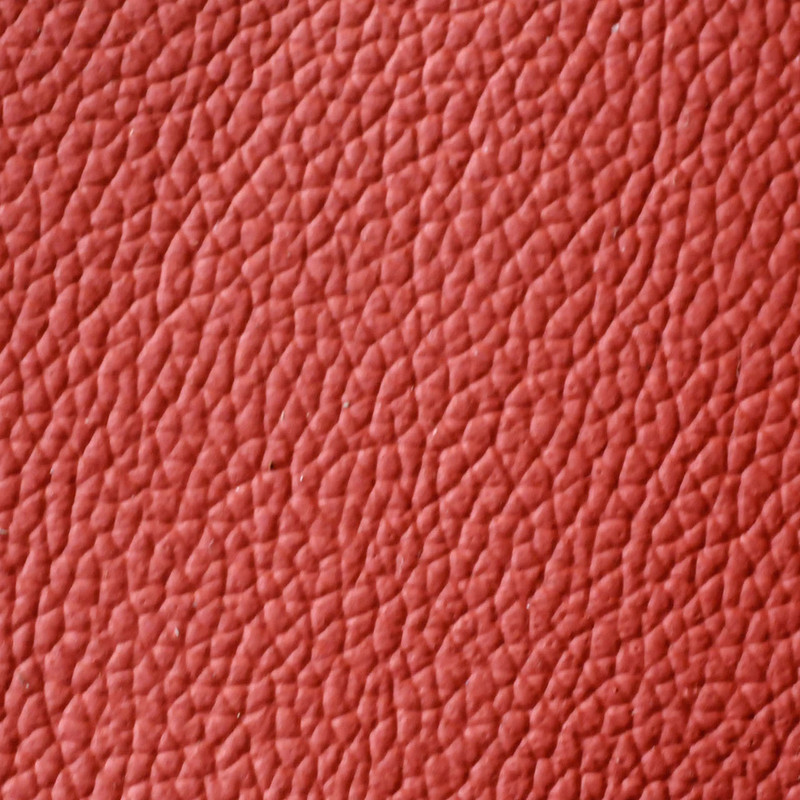This image is a highly detailed, zoomed-in macro shot, focusing on a brightly illuminated, richly textured surface. The photograph presents a close-up of what appears to be a sports ball, potentially a basketball evidenced by its rubbery, indented texture. The predominant color is a vivid, orangey-red, akin to a burnt orange or coral red. The surface is meticulously detailed, revealing intricate bumps and indents that suggest a tactile rubber or leather fabric. The image is well-lit, showing no prominent shadows, indicating that it was taken under strong daylight or artificial lighting. Some small irregularities, such as tiny bits of dirt and a few minor scratches, are noticeable on the surface, particularly in the center, which appears more focused and slightly shinier, likely due to the lighting emphasis. The lack of contextual elements and shadows directs full attention to the textured material itself, making it a captivating abstract representation.